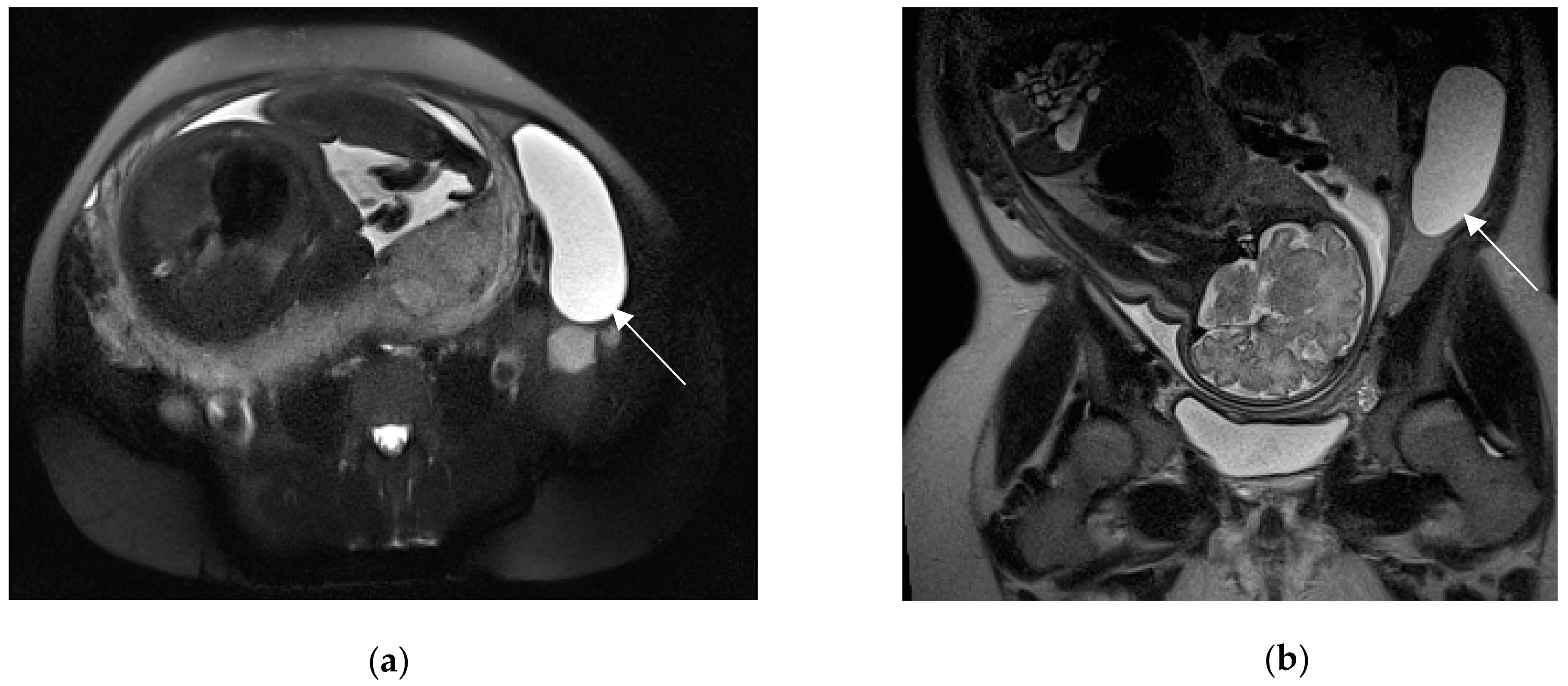The image depicts two black and white medical scans labeled (A) on the left and (B) on the right, separated by a white bar. Each scan features a white arrow pointing to a prominent, illuminated white structure inside the body, likely for scientific or medical study. Although the exact internal part is ambiguous, the targeted structure resembles a white kidney bean or oblong-shaped object. Both scans highlight this specific structure within a body, suggesting its significance in the examination. The remaining areas in the scans showcase various other internal structures, all presented in monochrome for detailed analysis.